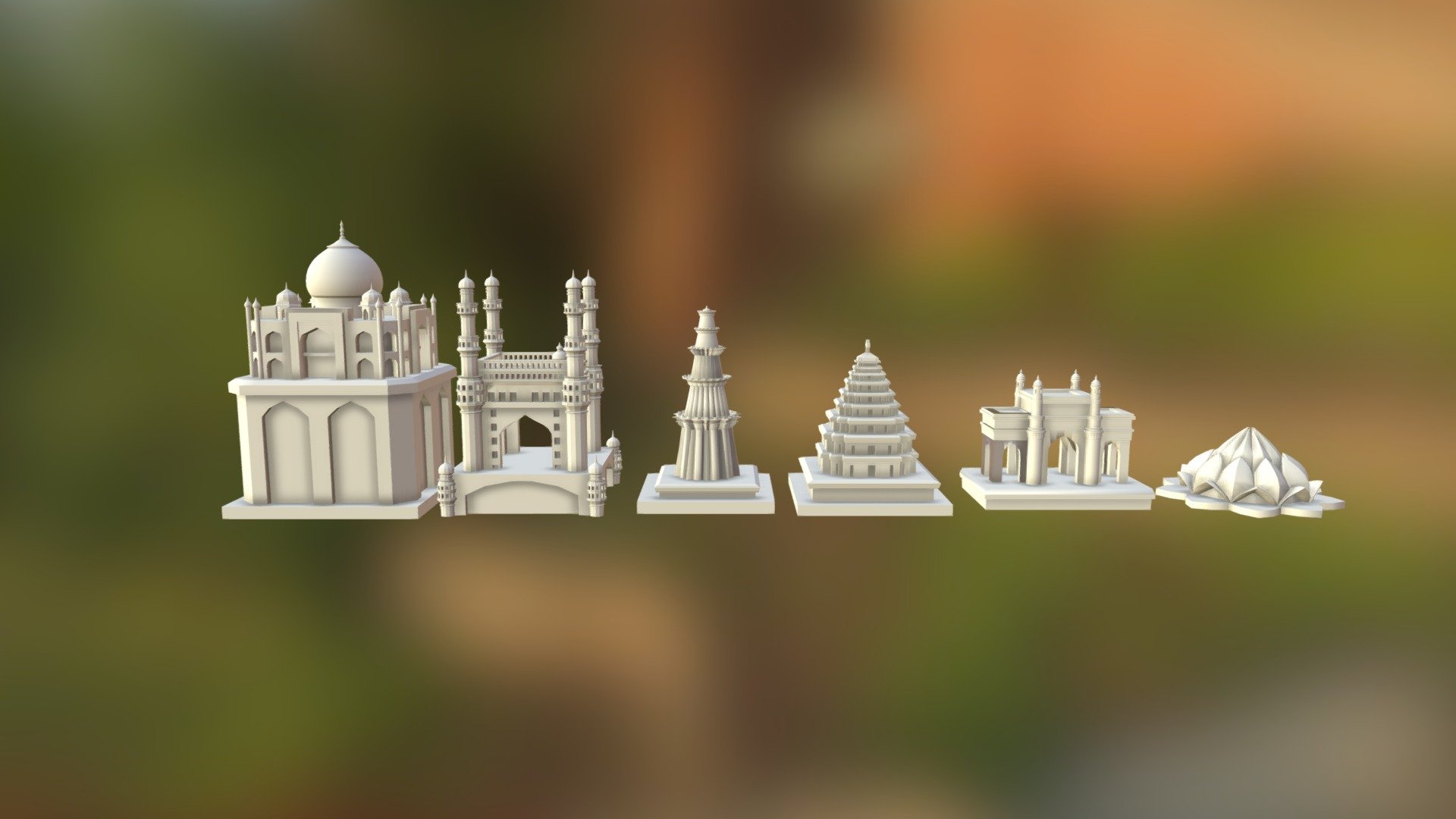A computer-generated image showcases six minimalistic, uncolored 3D renderings of famous temples, arranged horizontally in a descending order of size. The background is a blurred, predominantly green scene with touches of tan and orange. The structures, appearing as simplistic models, vary in form: On the far left is the largest, resembling the two-story Taj Mahal with a bulbous top. Next is a temple with four spires, followed by a spire-like building. Fourth in the sequence is a structure akin to a conical pyramid, next is a three-tiered Roman-style temple, and farthest right is a small mound, shaped like a collection of seashells or leaf formations. The temples, possibly representing different architectural styles around the world, are devoid of color and fine details, emphasizing their architectural forms in a minimalistic manner.